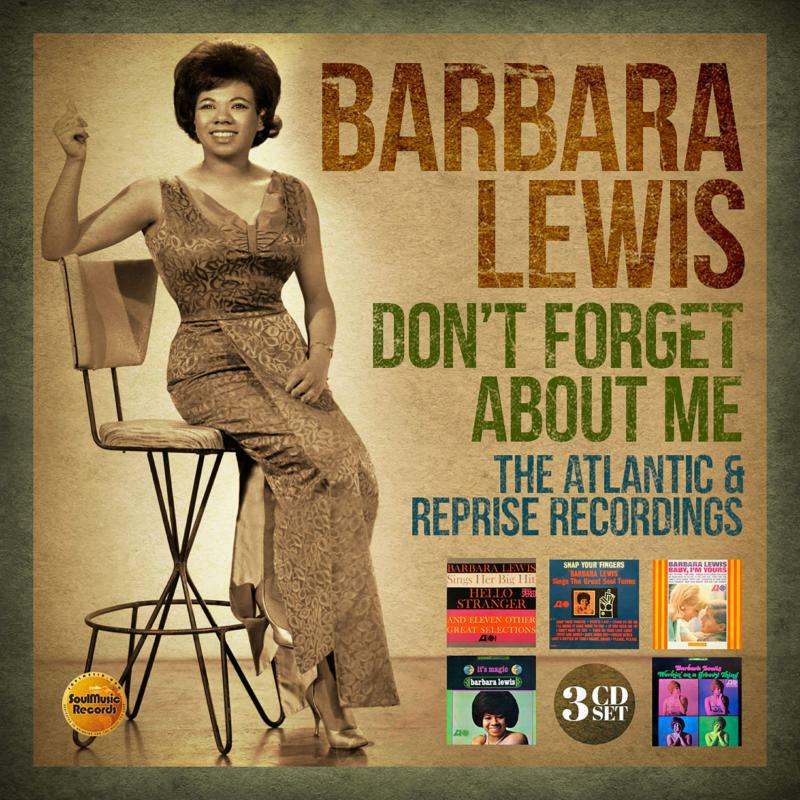The image is a detailed vintage poster featuring the cover of a music product by Barbara Lewis, framed in a green border. At the center is an African-American woman, Barbara Lewis, with a radiant smile, sitting on a long brown wooden chair with iron legs. She wears a sleeveless gown and golden-colored shoes, her dark hair cascading down. The backdrop consists of a light brown or yellow wall and a brown floor. 

The text beside her reads "Barbara Lewis, Don't Forget About Me" with her name in brown font and the title in green. Underneath, in dark blue, it states "The Atlantic and Reprise Recordings." An orange circular logo next to this text says "Soul Music Records."

At the bottom right-hand corner of the image, there are various CD covers displayed, and text indicating a "3 CD set" in white letters. Among the featured albums are "Hello Stranger and 11 other greatest collections," "Snap Your Fingers" with unclear text, "Baby I'm Yours" with a cover showcasing a man and a woman, "It's Magic, Barbara Lewis," and a CD cover segmented into four color zones, each featuring her image. The overall presentation blends a nostalgic aesthetic with detailed information about her music collection.